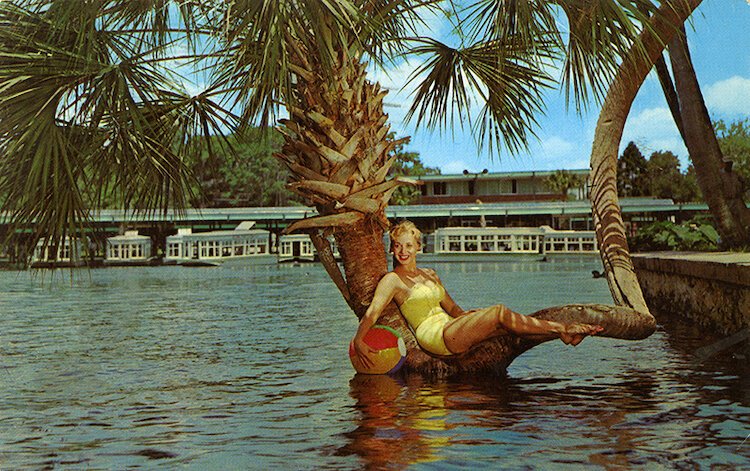In this captivating image, a blonde-haired woman with short hair and bright red lipstick is reclined on a uniquely twisted palm tree branch extending into dark, choppy water. She is wearing a vintage, canary yellow bikini and holds a vibrant beach ball with segments of red, yellow, green, blue, and a white top. The palm tree's canopy of leaves frames her head as she lounges with her legs outstretched and toes pointed. In the background, a clear blue sky with fluffy white clouds stretches over a landscape featuring a concrete shoreline, scattered tropical trees, and distant buildings with covered sections. A large building with an overhang and several smaller, sheltered structures can be seen near the water line, accompanied by boats docked at a pier behind her.